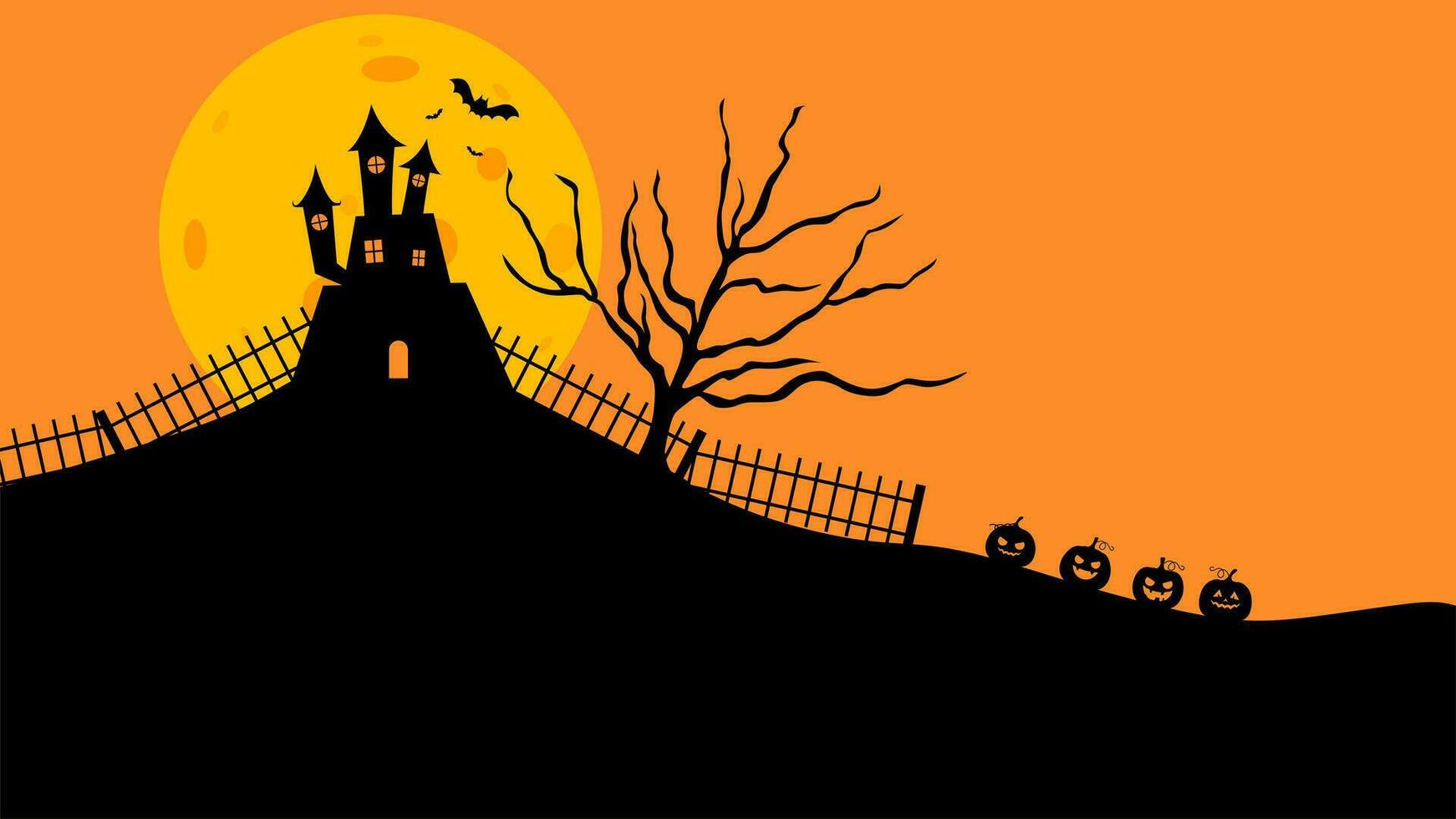This computer-generated Halloween-themed image features a horizontally aligned rectangular frame, predominantly colored in shades of orange and black. The background showcases a solid orange sky extending from the top to the middle of the image, symbolizing a spooky evening. Positioned on the upper left is a large, yellow moon with irregular cut-out shapes, adding to the eerie ambiance. In front of the moon stands a dark, imposing castle with three pointy, witch-hat-like roofs. 

To the upper right of the castle, three ominous bats are seen flitting through the orange sky. A black, gnarled fence stretches from either side of the castle, tracing the edge of a black hill that occupies the entire bottom portion of the picture. Perched on this hill, towards the right, are four black-shaded jack-o'-lanterns, their sinister faces illuminated in orange. A leafless, skeletal tree stands between the castle and the jack-o'-lanterns, enhancing the haunting atmosphere of this scene.